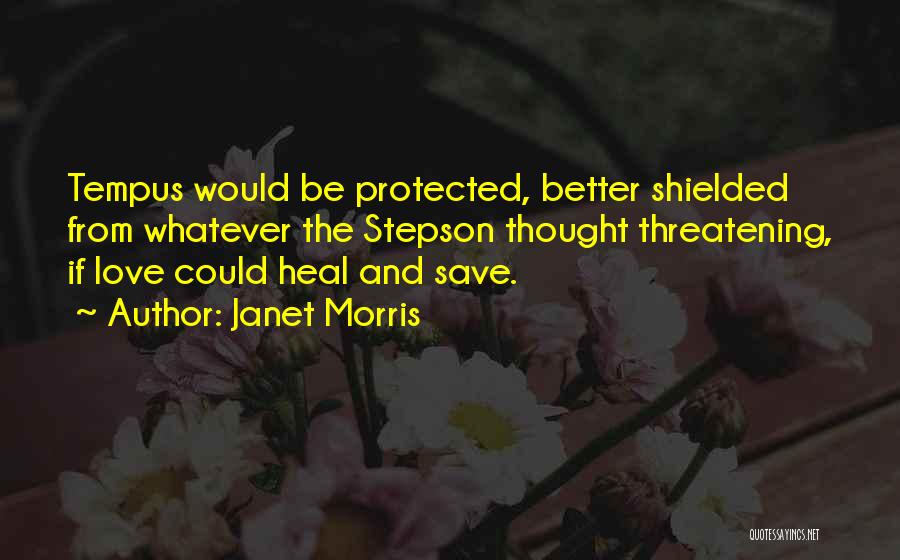The meme image features a dimly lit, dark photograph of a bouquet of flowers resting on a wooden table. The bouquet includes white and pink flowers with yellow centers, arranged on what appears to be a wooden surface, possibly a picnic table or a similar setting, with a faint glimpse of grass and a blurry, curvy black metal chair in the background.

Overlaying this floral background is a three-line quote in yellow text: "Tempest would be protected, better shielded from whatever the stepson thought threatening, if love could heal and save." The quote is attributed to Author Janet Morris, whose name appears beneath the quote. In the bottom right corner of the image, there is a small, white text that reads "quotesayings.net," denoting the source of the quote.